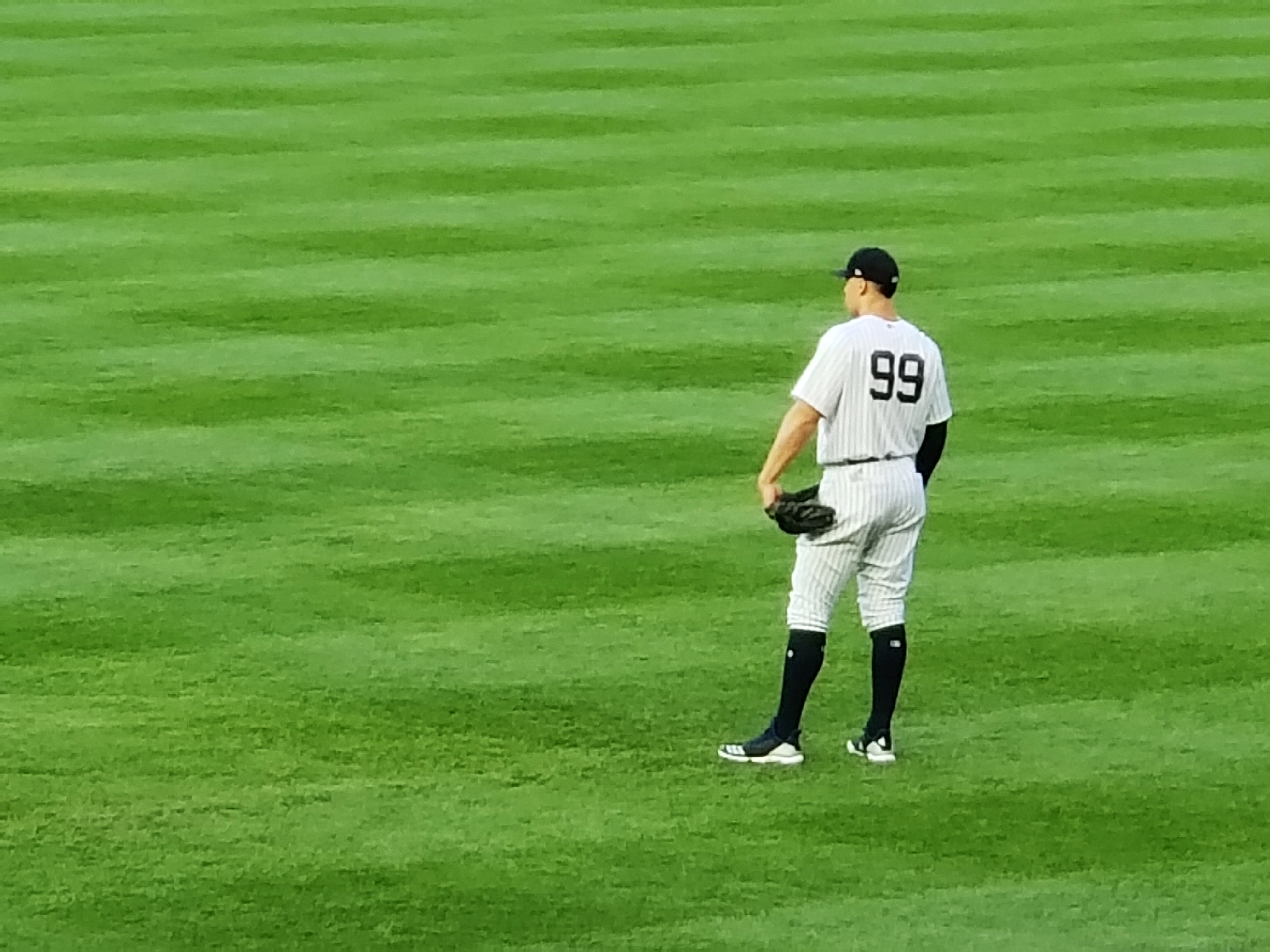This photograph captures baseball player Aaron Judge standing in the outfield, intensely watching the infield as though anticipating the play. Judge is clad in a white uniform with vertical black pinstripes, featuring the number 99 in bold black on his back. His ensemble includes a black baseball cap, tall black socks, black and white baseball shoes, and a black mitt in his left hand. He sports a short-sleeved jersey revealing his bare left arm, while his right arm appears dark, covered by a long-sleeved garment. The lush grass beneath him is meticulously mowed to create an eye-catching crisscross pattern of alternating dark and light green stripes, enhancing the visual appeal of the large, expansive field.